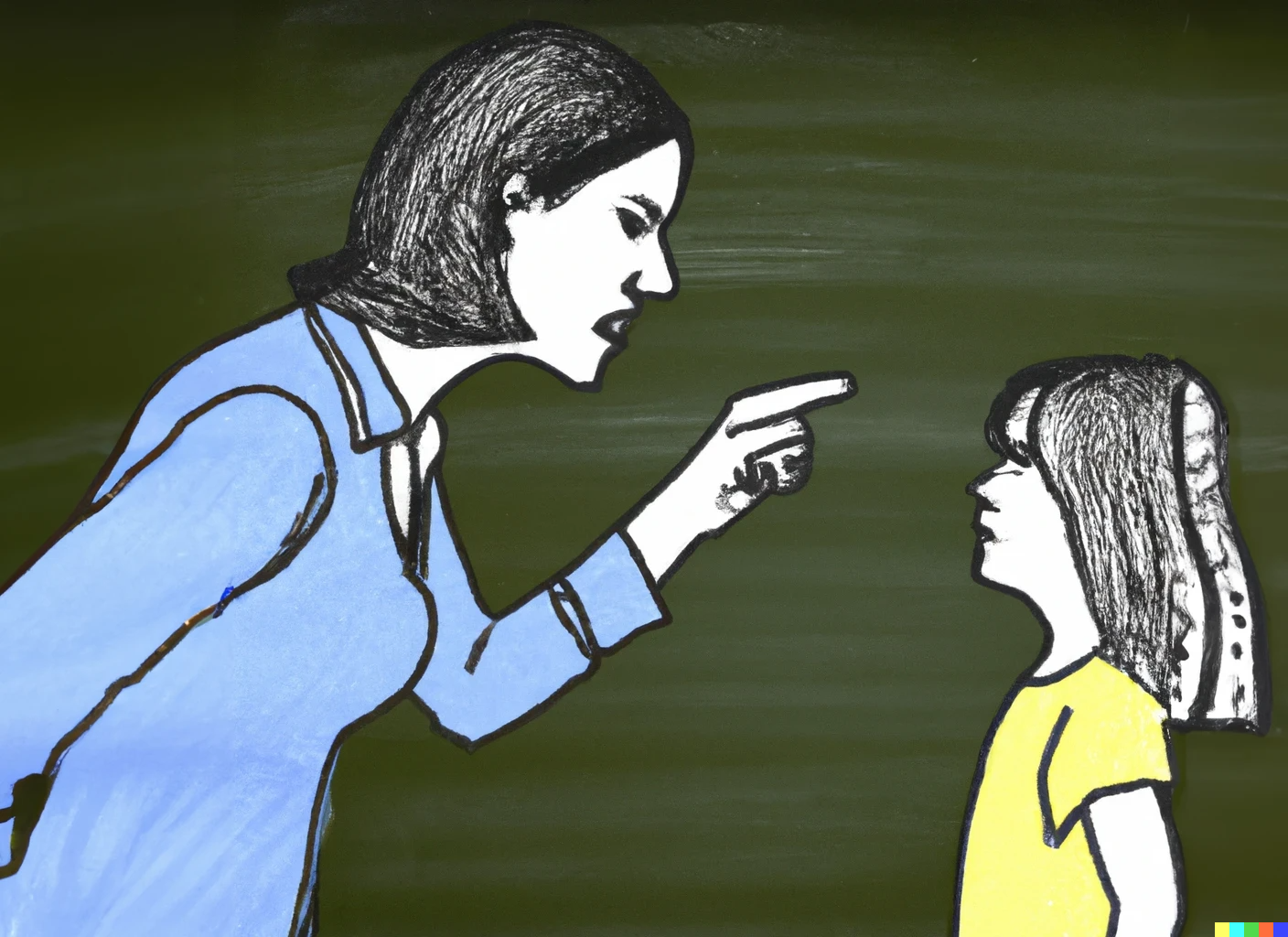This image appears to be a painting of an angry mother disciplining her young daughter. The artwork is housed within a wide vertical rectangular frame and features a dark green background composed of visible paintbrush strokes, giving it a textured, almost camouflage-like appearance. On the left side, the mother has short black hair styled into a bob, white skin with black outlines, and a blue long-sleeved blouse with a collar. Her expression is stern and angry, with her finger pointed accusingly at the child, one arm behind her back and the other bent at the elbow. The child, positioned on the right, has shoulder-length black hair with bangs, white skin, similarly outlined in black, and is wearing a short-sleeved yellow T-shirt. The child looks up at the mother with a stunned expression. In the bottom right corner of the image, there are small colored squares arranged sequentially in yellow, light blue, green, red, and either dark blue or purple, adding a touch of contrasting color detail. Each element in the image, from the brushstroke texture to the vivid expressions, works together to portray a tense moment of discipline between the mother and child.